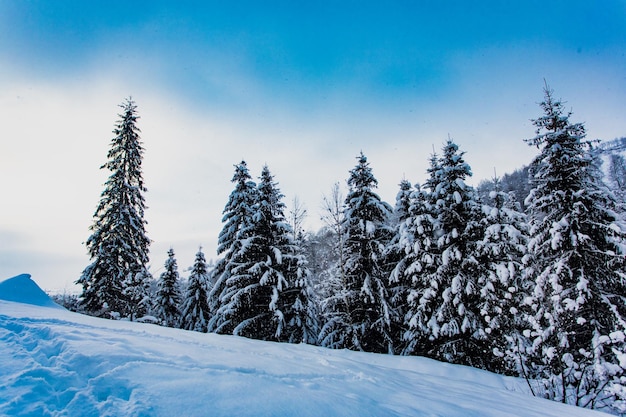This image captures a picturesque winter scene bathed in broad daylight. The ground is blanketed in deep, white snow, with a bluish tint in the bottom left corner where foot tracks meander in circular and straight patterns, indicating recent activity. Towering, dark green pines and shorter, leafless trees stand gracefully under a heavy cover of snow, their branches weighed down by the frosty accumulation. Some snow-covered sticks protrude from the ground, adding to the scene's intricate details. In the background, hilly terrain is dotted with more trees, providing a sense of depth and continuity. Above, the sky transitions from a clear, vibrant blue at the top to patches of white clouds or fog lingering in the midsection, enhancing the serene, cold beauty of the landscape.